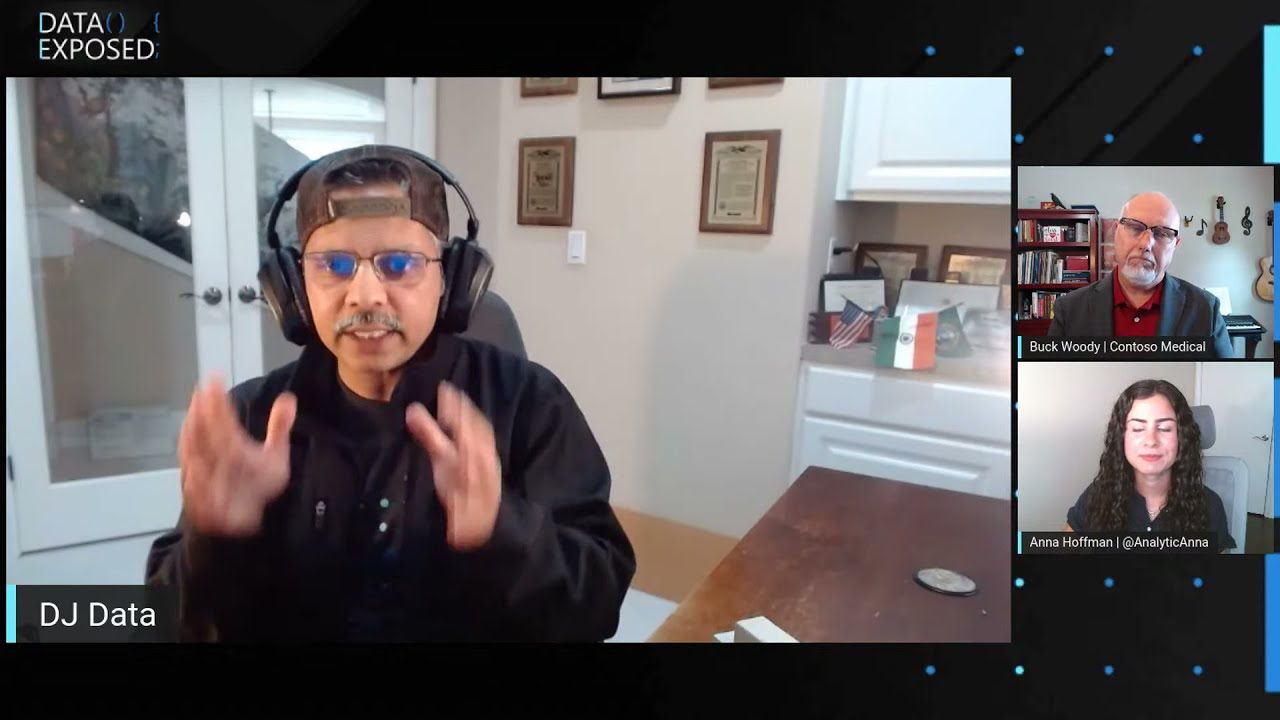The screenshot captures a dynamic Zoom meeting or podcast recording featuring three participants. The largest participant box on the left showcases the main host, DJ Data, an older male wearing glasses, a backwards baseball cap, a black long-sleeve shirt, and headphones. Behind him is a professional office setting with patio doors, white cabinets, a wooden desk, and multiple plaques on the wall. Notably, there's a display of country flags including an American Indian and Mexican flag.

On the right side, there are two smaller, stacked participant boxes. The top box features Buck Woody from Contoso Medical, identifiable by his short hair, glasses, gray jacket over a red shirt, and a gray beard. Surrounding him is a cozy office with guitars mounted on the wall, a bookcase filled with many books, and a generally warm ambiance.

The bottom box showcases Anna Hoffman, who has long curly black hair and wears a dark gray shirt. Her background is simpler, featuring a computer chair and a white door. The screen’s layout and the presence of "DATA EXPOSED" in white at the top left suggest that this is a podcast or show focusing on analytics or healthcare topics.